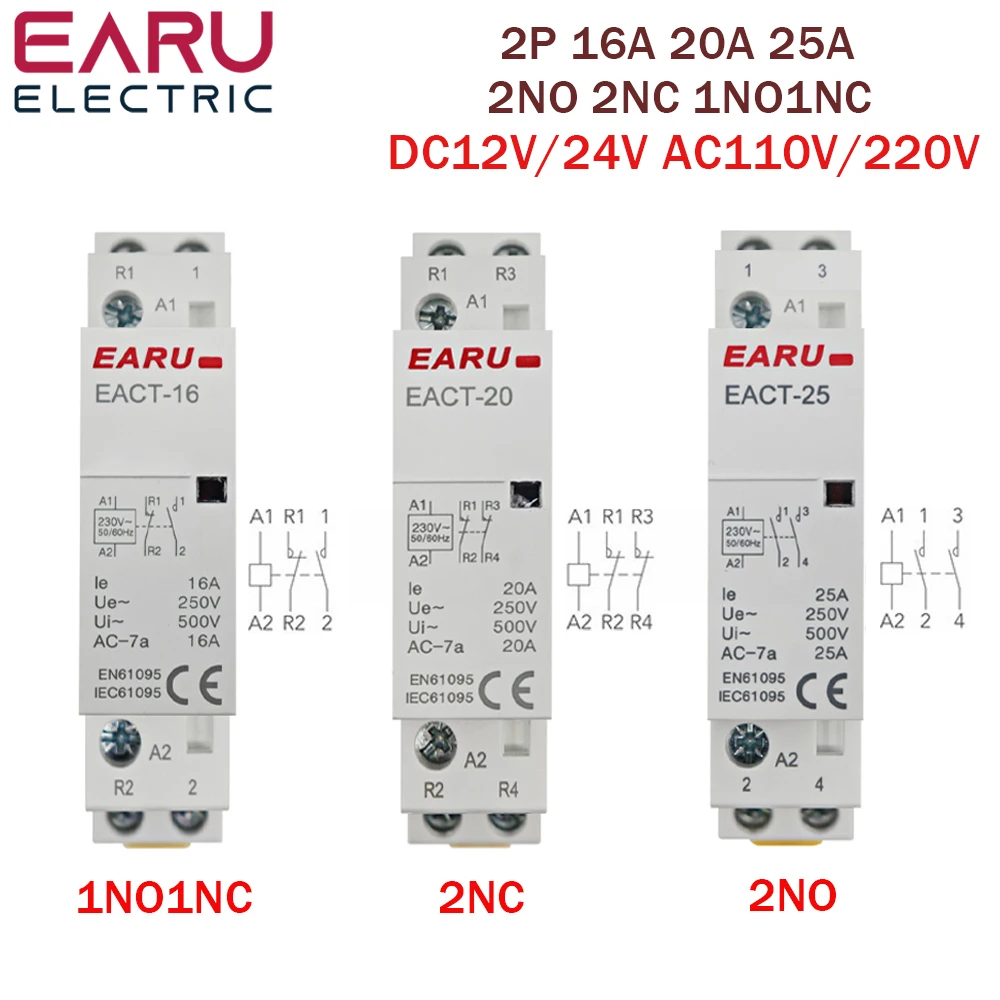The image depicts three electronic components, positioned side-by-side against a white background with equal spacing between them. Each component is labeled with the acronym "E A R U" in red at the top, where the "A" is stylized as an upside-down "V." Directly below this, in black, the word "electric" is displayed. Each component has a series of alphanumeric codes and specifications scattered across it, including "2P, 16A, 20A, 25A" and "2NO, 2NC, 1NO, 1NC," as well as voltage indicators like "DC 12V/24V" and "AC 110V/220V." Additionally, each component has smaller labels beneath them, with the first labeled "1NO 1NC," the second "2NC," and the third "2NO." The image contains colors such as black, gray, red, dark red, and silver. Despite the detailed text and intricate numeric codes, the precise function of these components remains unclear from the image alone.